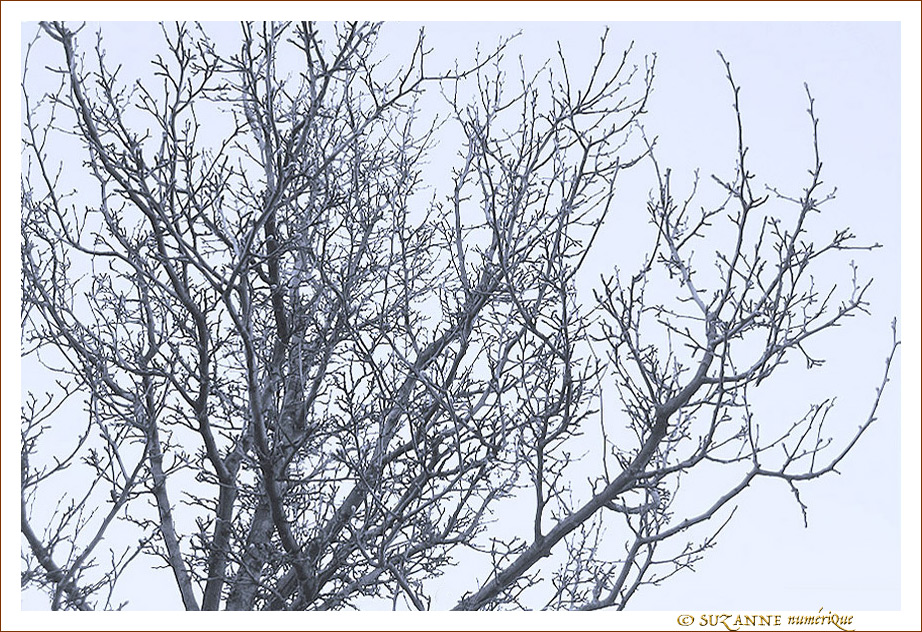This outdoor photograph, likely captured during the late winter or early spring, showcases the intricate details of a tall tree's upper branches against a predominantly gray sky, suggestive of a cold day. The tree itself is characterized by an abundance of bare branches and twigs, seemingly dormant but closer inspection reveals buds hinting at the onset of new growth, indicating the seasonal transition. In the bottom right corner of the image, a gold inscription reads "Suzanne Numerique N-U-M-E-R-I-Q-U-E" with a copyright symbol. The scene, viewed from a ground perspective looking up, is void of leaves or acorns, accentuating the stark, almost monochromatic contrast between the tree and the sky, which adds to the overall wintry feel of the photograph.